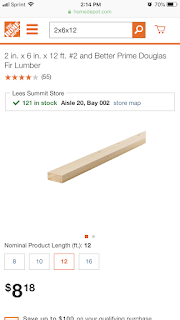The image is a screenshot of a website viewed on a smartphone. At the top center of the screen, the URL "homedepot.com" is displayed, with The Home Depot logo positioned in the upper left-hand corner. In the middle of the screen, there's a search bar where someone has entered "2x6x12." Towards the upper right corner, there's a shopping cart icon.

A specific product is shown below the search bar—titled "2 in. x 6 in. x 12 ft. #2 and Better Prime Douglas Fir Lumber." The product boasts a four-star rating based on 55 reviews. Information about availability is provided: "Lee's Summit Store, 121 in stock, Aisle 20, Bay 002," along with a button to view a store map.

The product image depicts a light-colored wooden plank. Underneath the image, a selection for product length is displayed, with options of 6, 10, 12, and 16 feet. The 12-foot option is highlighted. The price for this length is listed as $8.18.